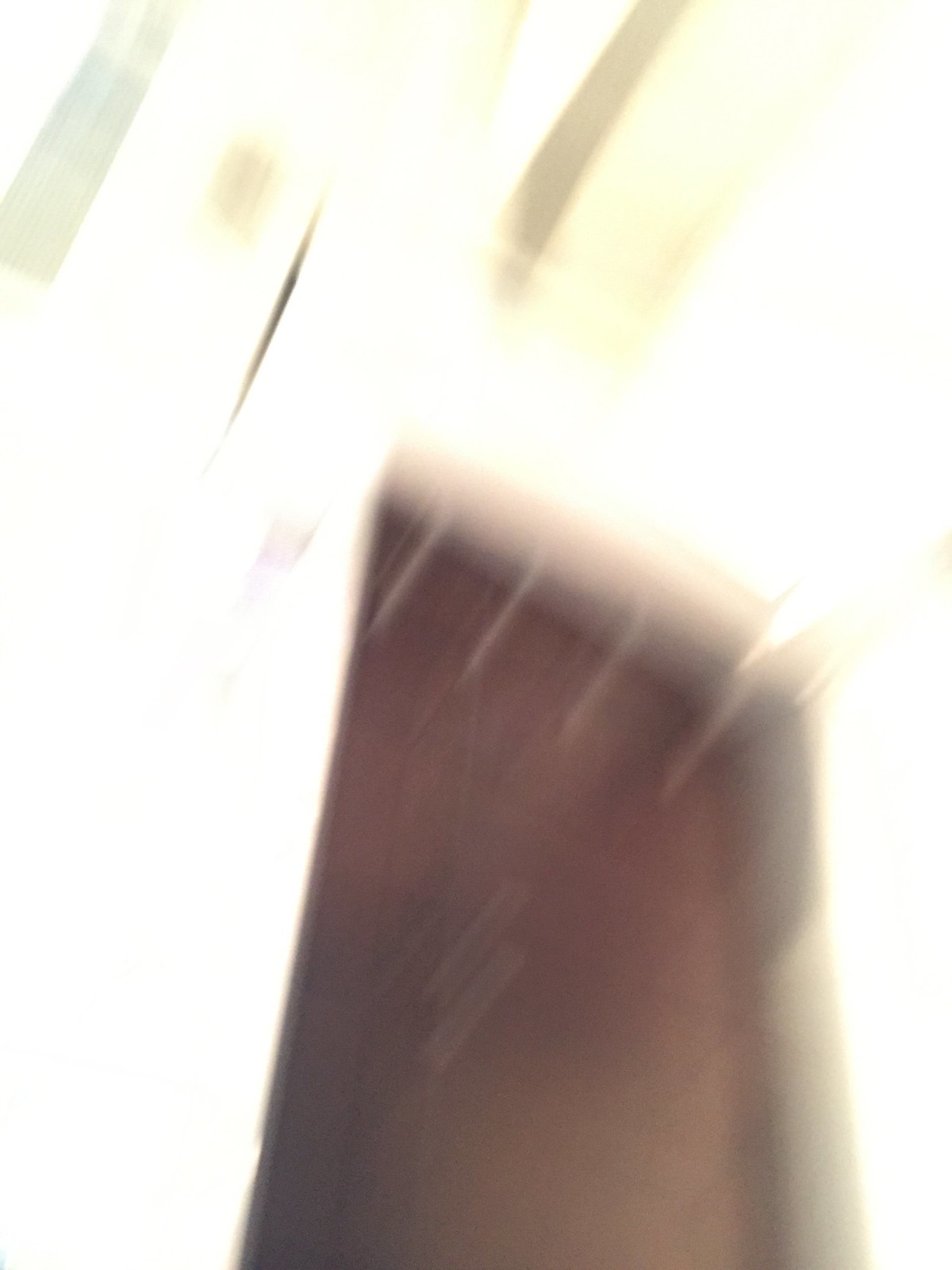A blurred image appears primarily white and seems to depict a vertically rectangular door with a white frame. The door itself appears brown, though it is obscured by the blur. Some indistinct lines emerge from the door, possibly artifacts of the camera motion or other elements within the frame. Above the door, there is a yellowish piece of wood, adding a contrasting hue to the predominantly monochromatic scene. To the upper left of this piece of wood, black lines are visible, contributing to the image’s complexity. Additionally, hanging down further to the upper left is another piece of wood, distinguishable by its whitish-gray color, adding an element of interest and texture to the composition.